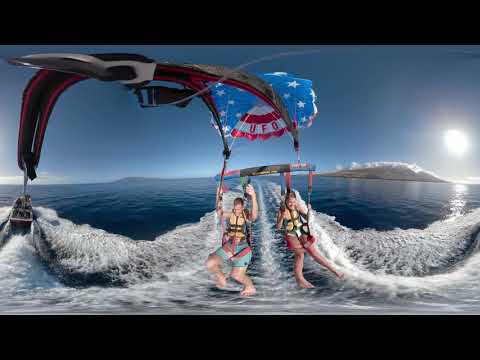In this vivid panoramic image, two teenagers, a boy and a girl, are joyfully parasailing above the open ocean waters. Their parasail, designed to resemble the American flag with red, white, and blue colors, prominently displays the word "UFO." They are barefoot, wearing life jackets, and kicking their feet up, splashing water as they are pulled by a modestly sized boat. The bright, sunny day contrasts with the snow-capped mountains in the background, creating a unique and almost surreal scene. The boat, facing away from the viewer, churns up frothy water visible beneath the parasailers and extends in arcs as part of the wake. A thick black border frames the top and bottom of this image, accentuating the panoramic view. The sun's glare can be seen slightly above the middle on the right side, adding a radiant effect to the ocean's wide expanse.